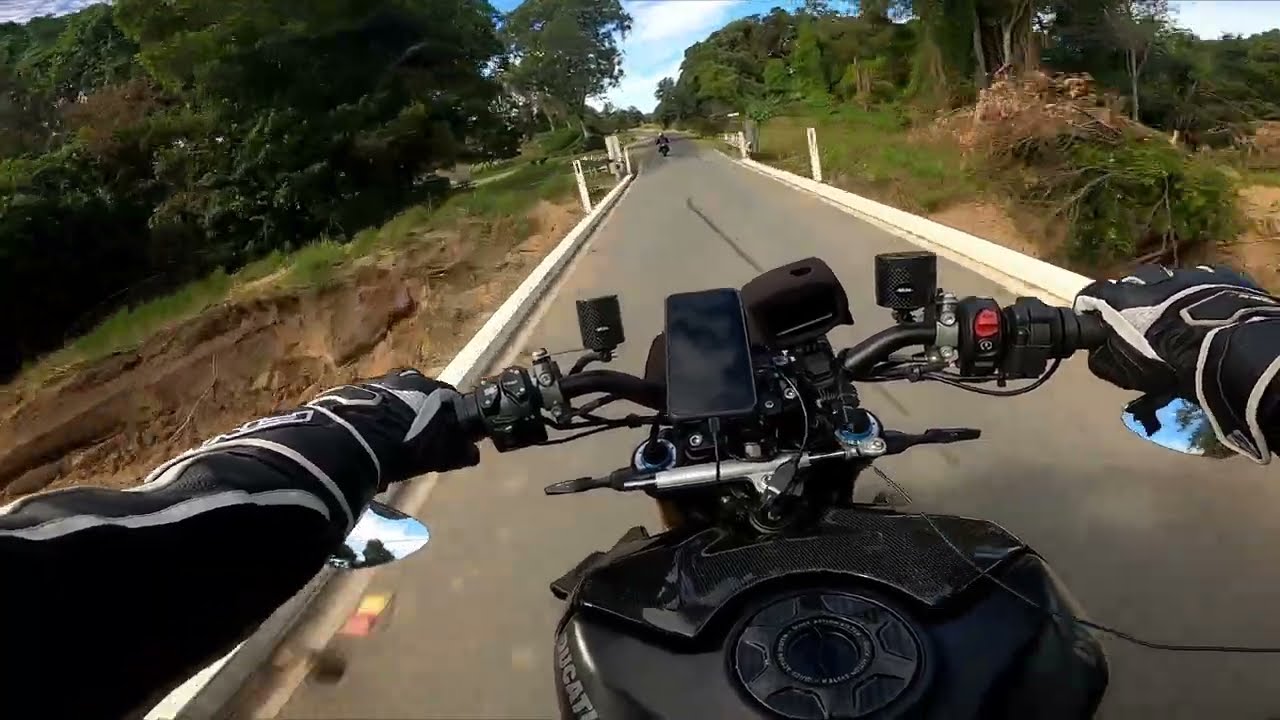The image presents a dynamic first-person perspective from a motorcyclist wearing a GoPro mounted on their helmet. The rider, clad in a black motorcycle jacket with white striping, has both hands firmly gripping the handlebars, adorned with matching black and white gloves. At the center of the motorcycle's handlebars, a smartphone is mounted and plugged in. The sleek black body of the motorcycle, which appears to be a Ducati, is prominent, with the gas tank cap visible below. The narrow street bridge they're traversing spans a ravine with dirt hills sloping down on either side, bordered by white barriers. The road ahead is paved, showing some motion blur, indicating the bike's speed. Further ahead, another motorcyclist can be seen, though details are indistinct, suggesting either pursuit or a shared journey. The scene is framed by a rural backdrop, with trees visible beyond the dirt hills.